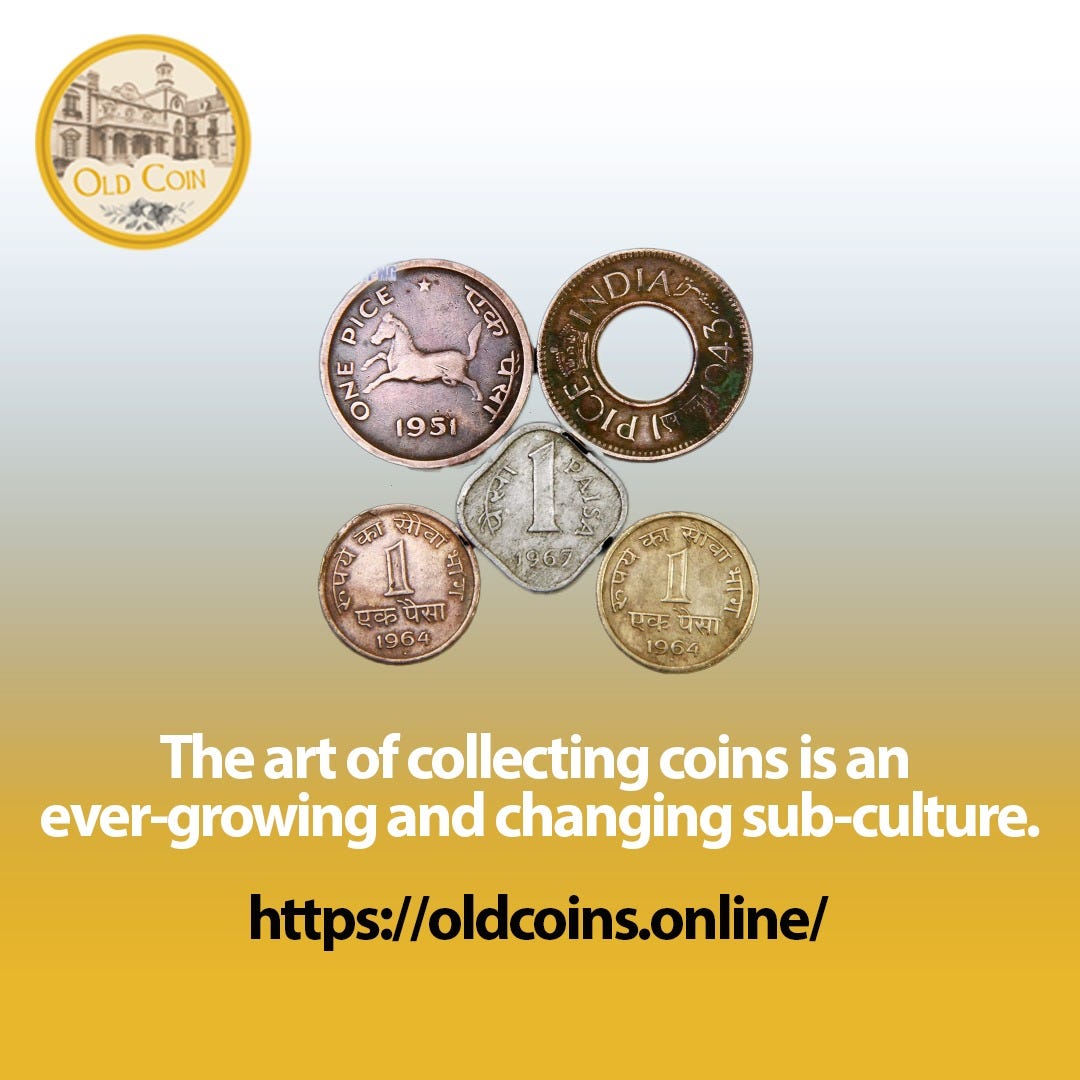The image features a collection of five coins arranged over a light white and blue background with a green bottom and blue center. The coins display various designs and dates, including a solid coin with a horse from 1951 labeled "one pice," an Indian coin with a hole in the center from 1943, and a square coin with rounded corners from 1967. There are also smaller coins, one of which is from 1964. In the upper left corner, there is a circular emblem with a building and the text "Ocoin." At the bottom, white text reads, "The art of collecting coins is an ever-growing and changing subculture," with the website "ocoins.online" in black text underneath.